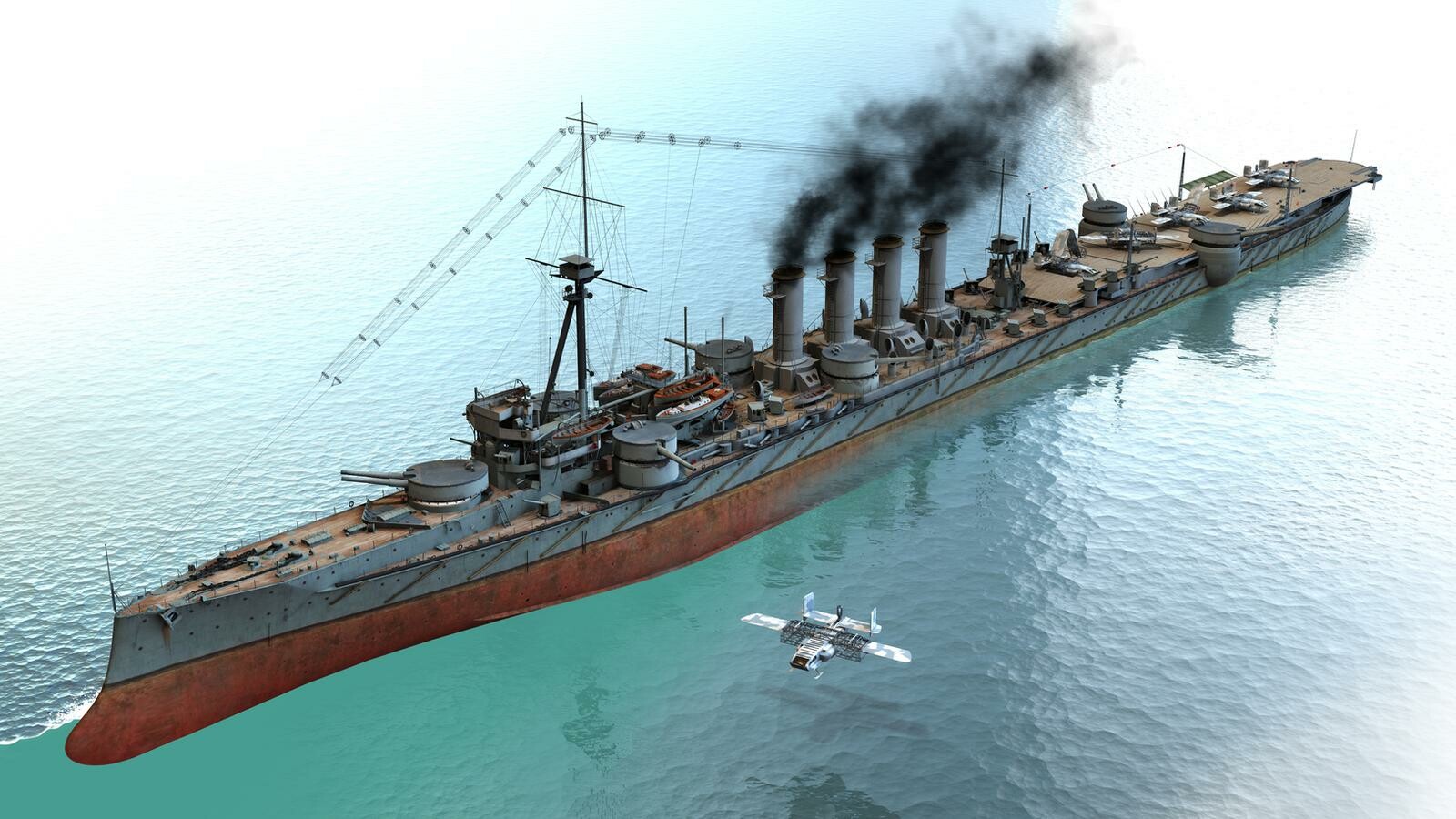The image depicts a highly detailed, computer-generated battleship, reminiscent of a scene from a video game, navigating a blue-green ocean. The ship, with a striking contrast of a red hull at the bottom transitioning to a gray superstructure, appears long and sleek with a narrow build. Dominating the midsection of the vessel are four smokestacks, each emitting thick black smoke that trails past the intricate network of wires extending from the bow to the stern. Situated on the forecastle is a prominent radio tower, surrounded by various metal and wooden posts, all linked by a web of ropes and cables. The deck bristles with several gun turrets, adding to its formidable appearance. At the stern, there are five stationary warplanes, and a sixth plane can be seen flying off to the port side, hinting at the ship's readiness for combat. On the starboard side, a light source illuminates the vessel, casting sharp highlights and shadows. Additionally, a drone hovers near the ship, enhancing the modernity of this digital artwork.